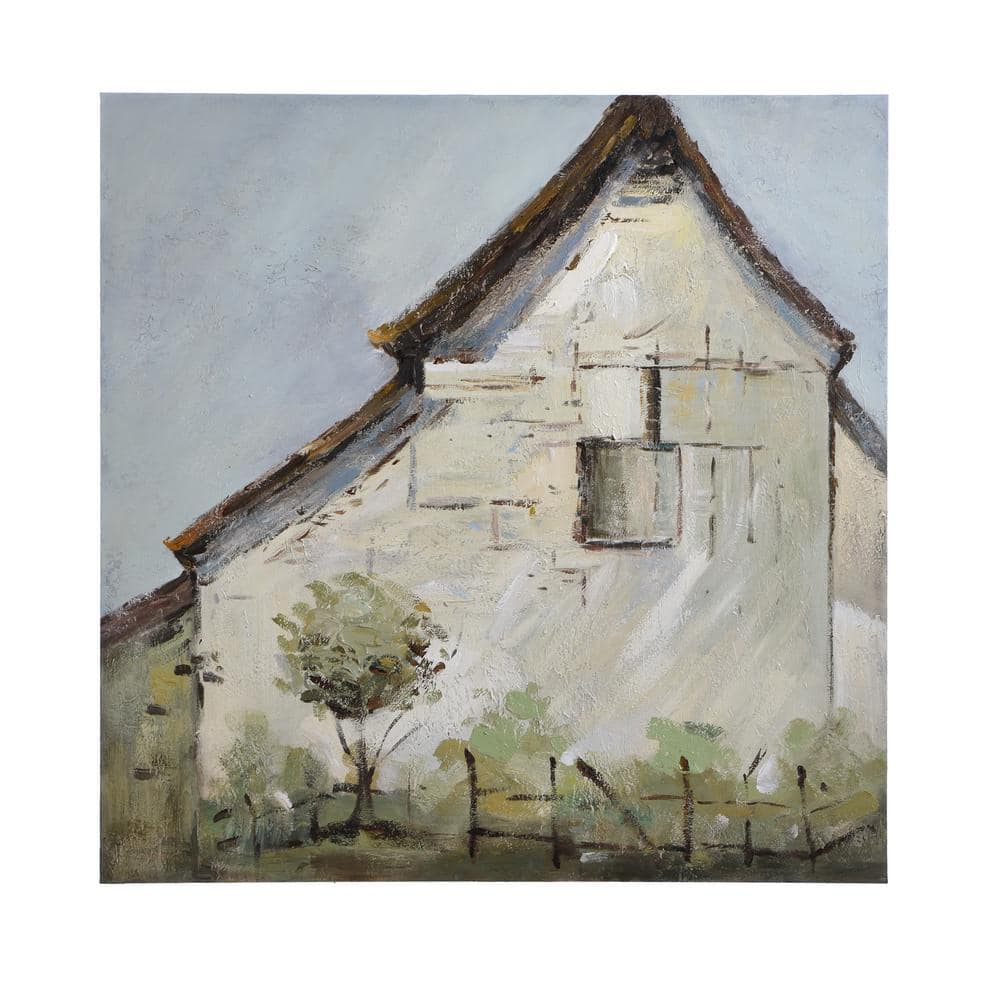This abstract painting features a modest, cream-colored house with hints of light green and blue, accentuated by soft white and gray brush strokes. Although the roof is brown and triangular, only the edges are visible. Below the roof, a light blue border adds subtle detail. The house features a single gray window positioned centrally on its side. In the foreground, a brown wooden fence, appearing somewhat broken, encloses the property. The bottom of the painting depicts green bushes and a short tree with a circular green top, suggesting leaves. The sky above is a muted grayish blue, devoid of distinct clouds, blending seamlessly with the overall tranquil and understated color palette.